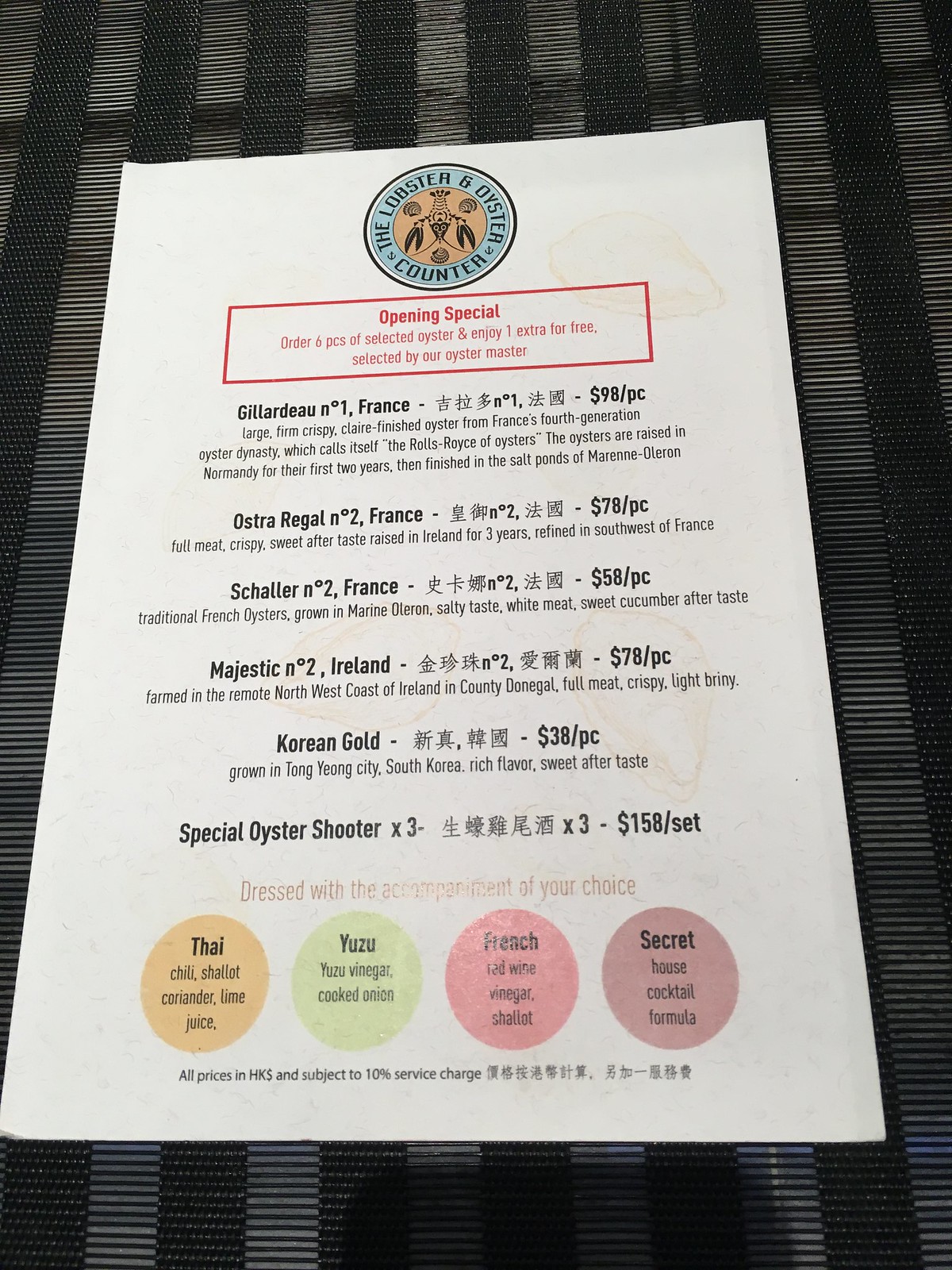**Menu Description for "The Lobster and Oyster Counter"**

At the top of a pristine white menu, elegantly placed on a sophisticated gray-black tablecloth, the title "The Lobster and Oyster Counter" is prominently displayed. Centered just below the title, a circular logo showcases an intricate drawing of a lobster, emphasizing the seafood-centric offerings of this establishment.

Highlighted in bold red text, an "Opening Special" is advertised within a striking red and white triangular emblem. While the detailed text of the instructions is unreadable, the visual cue commands attention.

Beneath this, a list of gourmet oyster options is meticulously detailed:
- **Guillardeau, France:** $98 per piece, accompanied by ingredients that are indecipherable but suggest exclusivity.
- **Ostra Regal No. 2, France:** $78 per piece, promising a royal taste experience.
- **Schaller, France:** $58 per piece, labeled with a unique "Schaller S-C-H-A-L-L-E-R" and curious "two degrees" specification.
- **Korean Gold:** $38 per piece, renowned for its exotic appeal.
- **Special Oyster Shooter:** $150 per set, hinting at an extravagant, indulgent tasting experience.

At the bottom, a series of circular images represent different oyster varieties and their origins:
- **Thai:** Suggesting a hint of Asian culinary influence.
- **Uzi:** Potentially a rare or secretive offering.
- **French:** Indicating a classic and refined choice.
- **Secret:** Mysteriously teasing an exclusive selection.

All these elements collectively create a sophisticated and enticing overview of "The Lobster and Oyster Counter," hinting at a culinary adventure that awaits diners at this elegant restaurant.